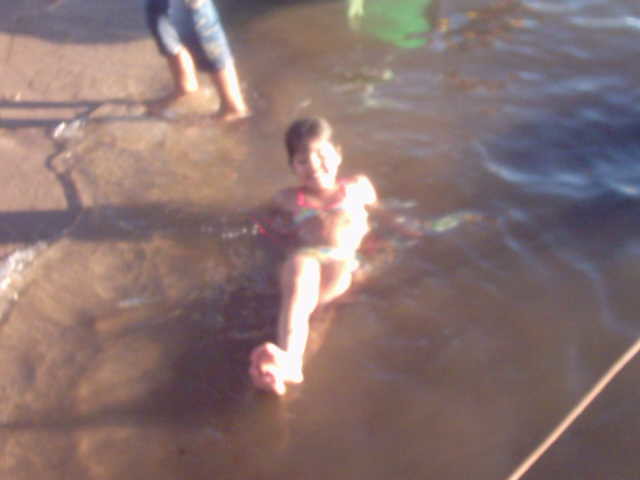A blurry photograph captures a joyful moment of a young child lying on their back in shallow, brackish water at the edge of a beach. The child, donned in a vibrant blue and pink two-piece swimsuit and arm floaties, smiles brightly while partially submerged in water. The sandy shore beneath them appears wet and muddy. Another figure, only visible from the knees down, stands in the water behind the child, wearing torn blue jeans that reach mid-calf. A string runs from the bottom right of the image to the side, adding to the sense of a casual, candid scene. The overall image focuses on the playful interaction with the shallow tide and the serene, carefree moment of the child.